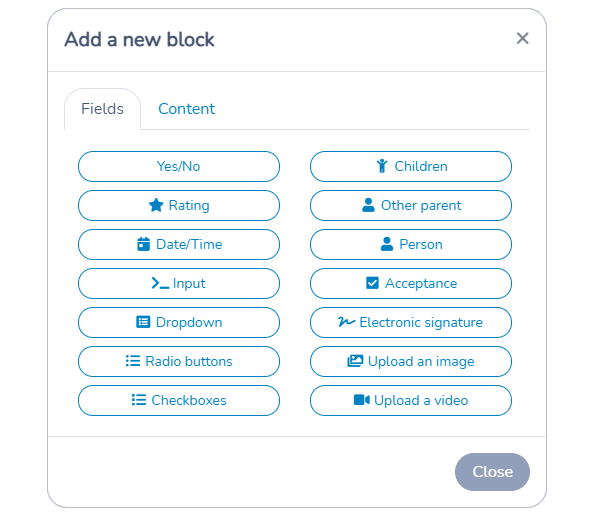The image is a screenshot of a selection interface. At the top left, it features an option labeled "Add a New Block." Positioned beneath this label, towards the bottom left, there are two tabs: "Fields" and "Content." The current active tab is the "Fields" tab. 

Within the "Fields" tab, there are two columns displaying a variety of options. The left column, listed from top to bottom, includes the following options: 
- Yes/No
- Rating
- Date/Time
- Input
- Drop Down
- Radio Buttons
- Checkboxes

The right column, also listed from top to bottom, presents these options:
- Children
- Other Parent
- Person
- Acceptance
- Electronic Signature
- Upload an Image
- Upload a Video

At the very bottom of the interface, there is a "Close" button, indicating the option to exit the selection interface.